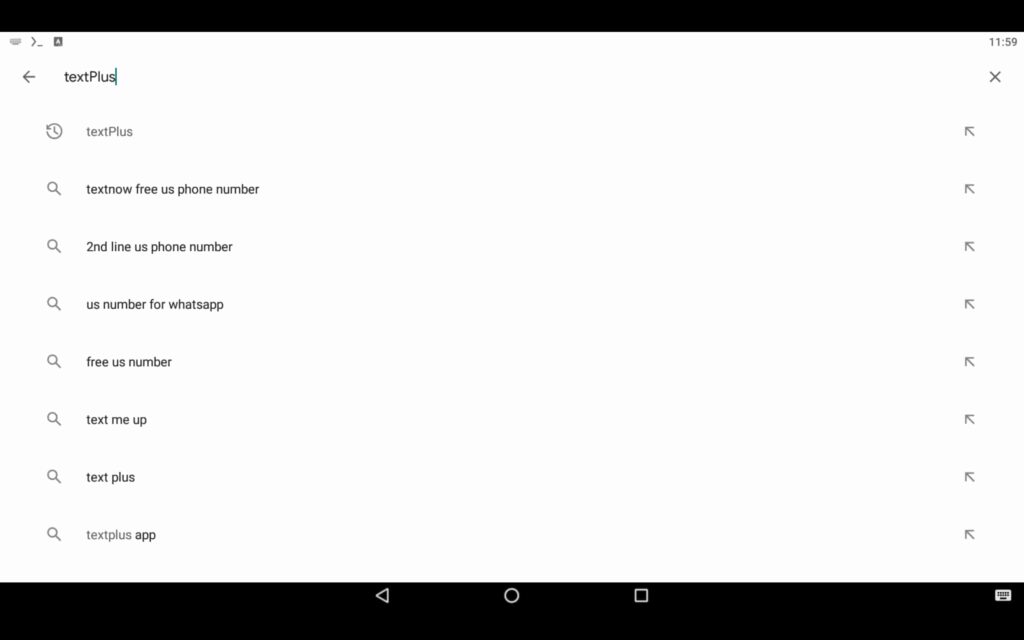The image features a stark white background with a black strip running horizontally across both the top and bottom. In the top right corner of the black strip at the top, the time is displayed as "11:59." On the top left-hand side, there's a gray or black arrow pointing left, next to the text "TextPlus," with a green line immediately following the "S." Below this, the phrase "TextPlus" is repeated in gray, followed by "TextNow" in black. The subsequent text underneath these includes the phrases "Free US Phone Number," "US Phone Number for WhatsApp," "Free US Number," "Text Me Up," another instance of "TextPlus," and finally, "TextPlus App."

On the left-hand edge of the image, next to each line of text, there is a small search icon (magnifying glass symbol). On the right-hand side, just below where the time "11:59" is displayed, there is a small "X" symbol. Adjacent to each line of text on the right side, there is an upward-pointing arrow tilted slightly to the left, indicating some form of navigation or highlighting option for each category listed.